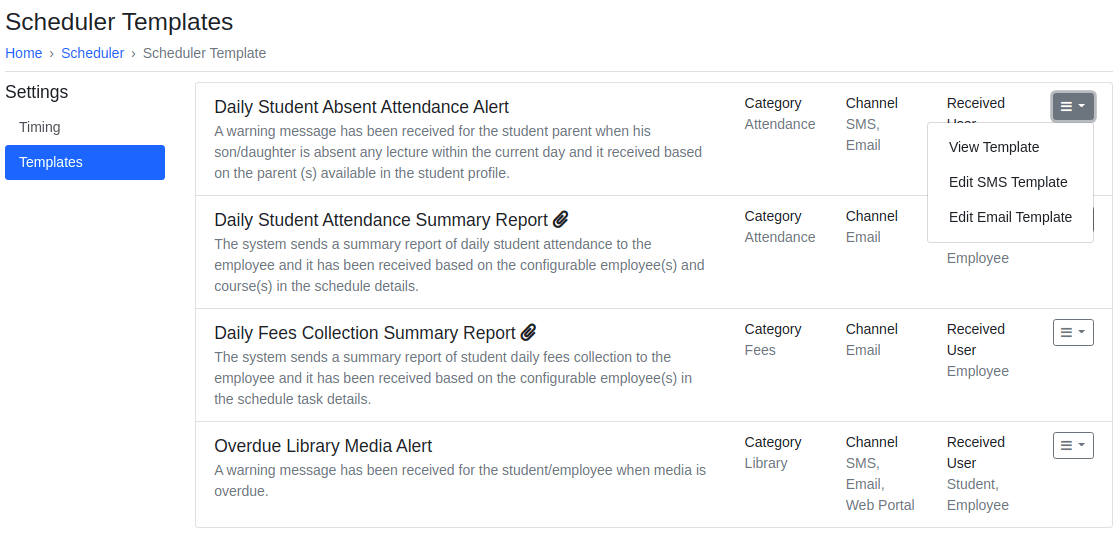The image displays a detailed interface of a scheduling and alert system, set against a clean white background. 

In the top left corner, there's a header labeled "Scheduler Templates." Below it, a navigation breadcrumb trail in blue text reads: "Home > Scheduler > Scheduler Template." Further down, there's a Settings menu with two options: "Timing" and "Templates," the latter of which is highlighted in blue.

Centered on the right side are four alert titles stacked vertically:
1. **Daily Student Absent Attendance Alert**
2. **Daily Student Attendance Summary Report**
3. **Daily Fees Collection Summary Report**
4. **Overdue Library Media Alert**

Each title is accompanied by a brief descriptive text underneath.

To the right of these titles, several columns - Category, Channel, and Received - organize pertinent details. The categories listed are as follows:
- Attendance
- Attendance
- Fees
- Library

The channels through which alerts are sent are listed in the Channel column:
- SMS, Email
- Email
- Email
- SMS, Email, Web Portal

In the Received column, a pop-up obscures the first row, offering three options: "View Template," "Edit SMS Template," and "Edit Email Template." The subsequent rows are labeled "Employee," "Received User Employee," and at the bottom, "Student and Employee."

Overall, the interface provides an organized and accessible layout for managing scheduling templates and related alerts.